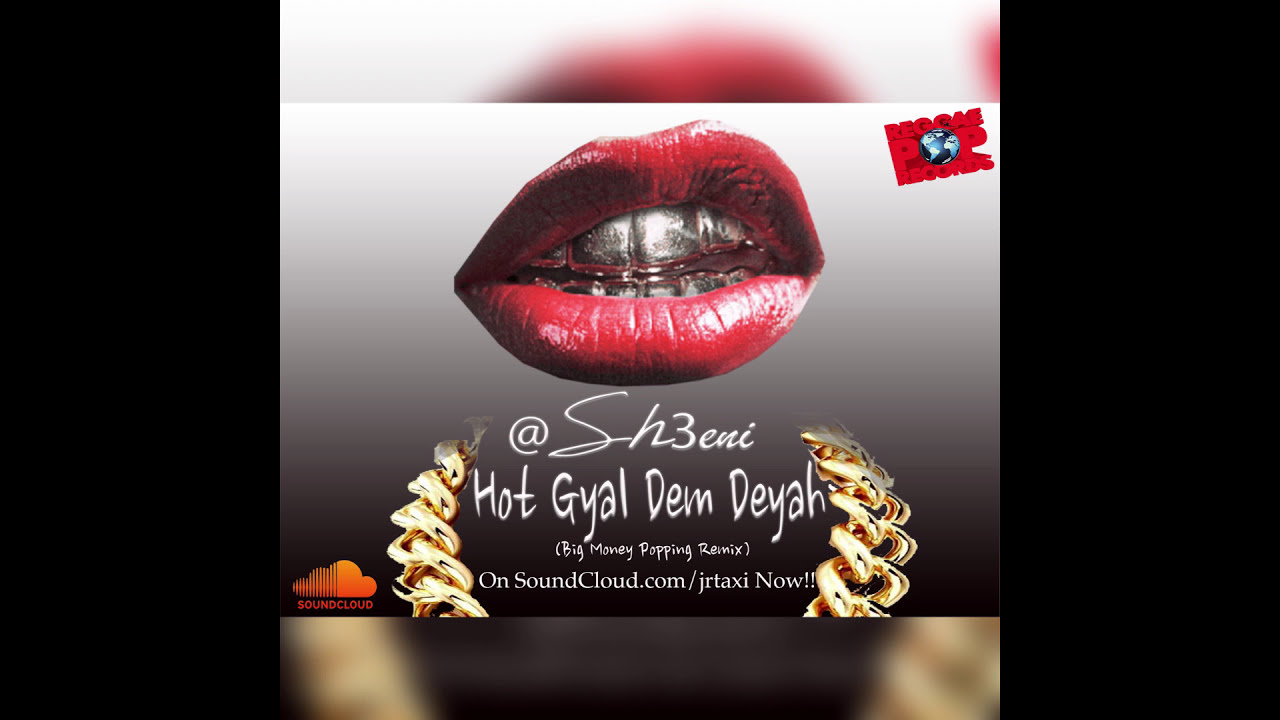The image is an advertisement for a new music release on SoundCloud. Dominating the top center are striking red lips, adorned with a gold grill on the teeth, flanked by segments of a gold chain on either side. The background elegantly fades from gray to black, enhancing the vibrancy of the colors. In the top-right corner, the logo for Reggae Pop Records is prominently displayed in red, featuring an earth symbol that adds hints of green and blue. Beneath the lips, the text reads: "@SH3ENI Hot Gyal Demdaya Big Money Popping Remix" in white, followed by "on soundcloud.com/JRTaxi now!!". The bottom left corner showcases the SoundCloud logo in its signature orange. This captivating and detailed composition effectively advertises the new album available on SoundCloud.